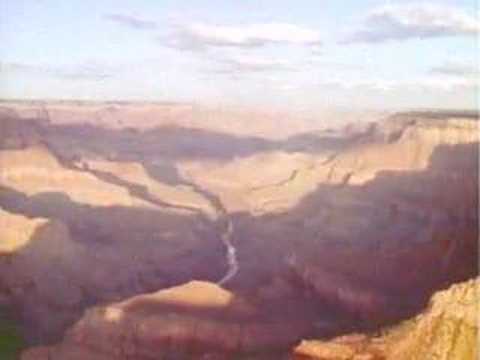The photograph captures a vast section of a canyon, likely the Grand Canyon, enveloped in deep and expansive shadows cast by clouds drifting above. The canyon’s interior features rugged, tan-colored walls that transition into darker shades of brown towards the center, suggesting depth and complexity. The image is somewhat out of focus, giving it a soft, almost ethereal quality. Dominating the sky are a few large, fluffy white clouds against a light blue backdrop, with no indication of impending bad weather. Towards the bottom center of the image, the meandering path of what appears to be the Colorado River is faintly visible, partially hidden by the prominent shadows that cloak the front of the canyon. This scenic view, encompassing three-quarters of the photo, provides a detailed and immersive glimpse into the majestic and storied landscape.